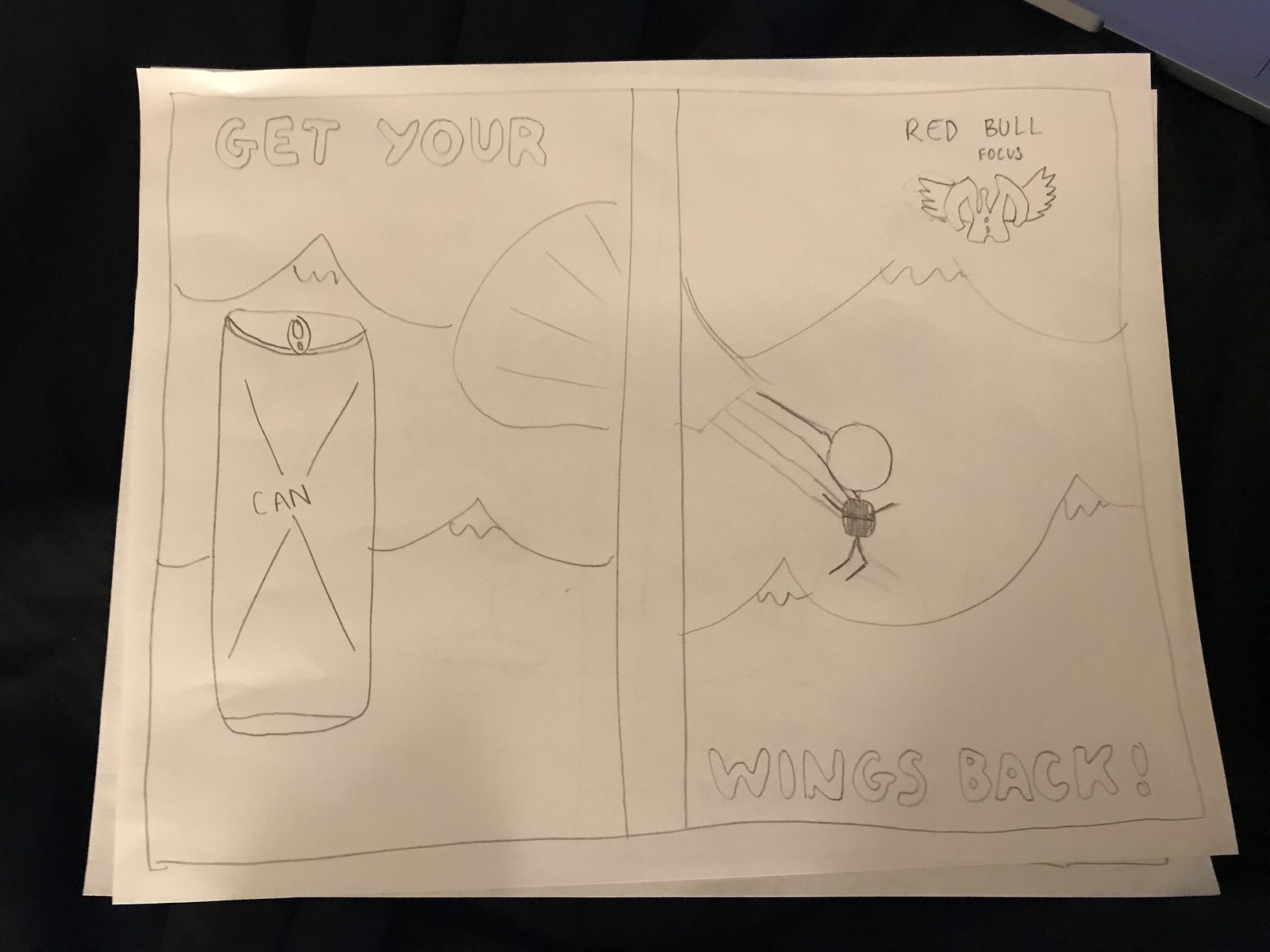This is a photograph of a child's pencil sketch on a white piece of paper set against a black tabletop, depicting a two-panel comic styled as a Red Bull advertisement. In the left panel, a vertical rectangle showcases the phrase "Get your" in bubble letters at the top, with an aluminum can labeled "can" and marked with an X slightly to the right. A portion of a curved "C" hinting at a parachute is also visible. The right panel continues this imagery with the phrase "wings back" in bubble letters at the bottom. A stick figure equipped with a parachute and backpack appears at the center, skydiving over a backdrop of mountains. In the lower right corner of the right panel, there's a Red Bull logo or icon, emphasizing the brand focus. The entire sketch is monochromatic, created with pencil on paper.